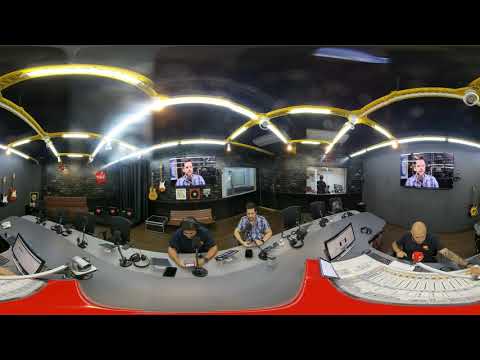This is a panoramic photograph capturing a detailed scene inside what seems to be a music or television studio, perhaps a control room. The image is slightly distorted, possibly indicating it was taken from a security camera with a letterbox format, featuring black rectangles on the top and bottom of the photo. In the foreground, we observe a long grey countertop with red accents, around which several men are seated.

At the center of the scene, two men with brown hair are seated at the desk, which also holds numerous microphones—around eight to ten in total. Behind them is a wall adorned with hanging guitars and large screen TVs. On these screens, a live image of a man’s head and shoulders is being projected. One of these men appears to be speaking into a microphone and wearing earphones, suggesting they are anchoring or managing a production.

To the right, a man in a white t-shirt with blonde hair is positioned at a white control panel or mixing board, with a computer monitor next to him. This panel, described as an equalizer measuring board, is likely used to control various sound inputs for the studio.

The studio’s ceiling is black and features fluorescent tube lights mounted on yellow rafters or beams. The room is windowless, illuminated by strategic lighting on the walls, enhancing the control room atmosphere. Overall, the photo captures a bustling scene of coordination and production, meticulously detailing the environment and roles of the individuals present.